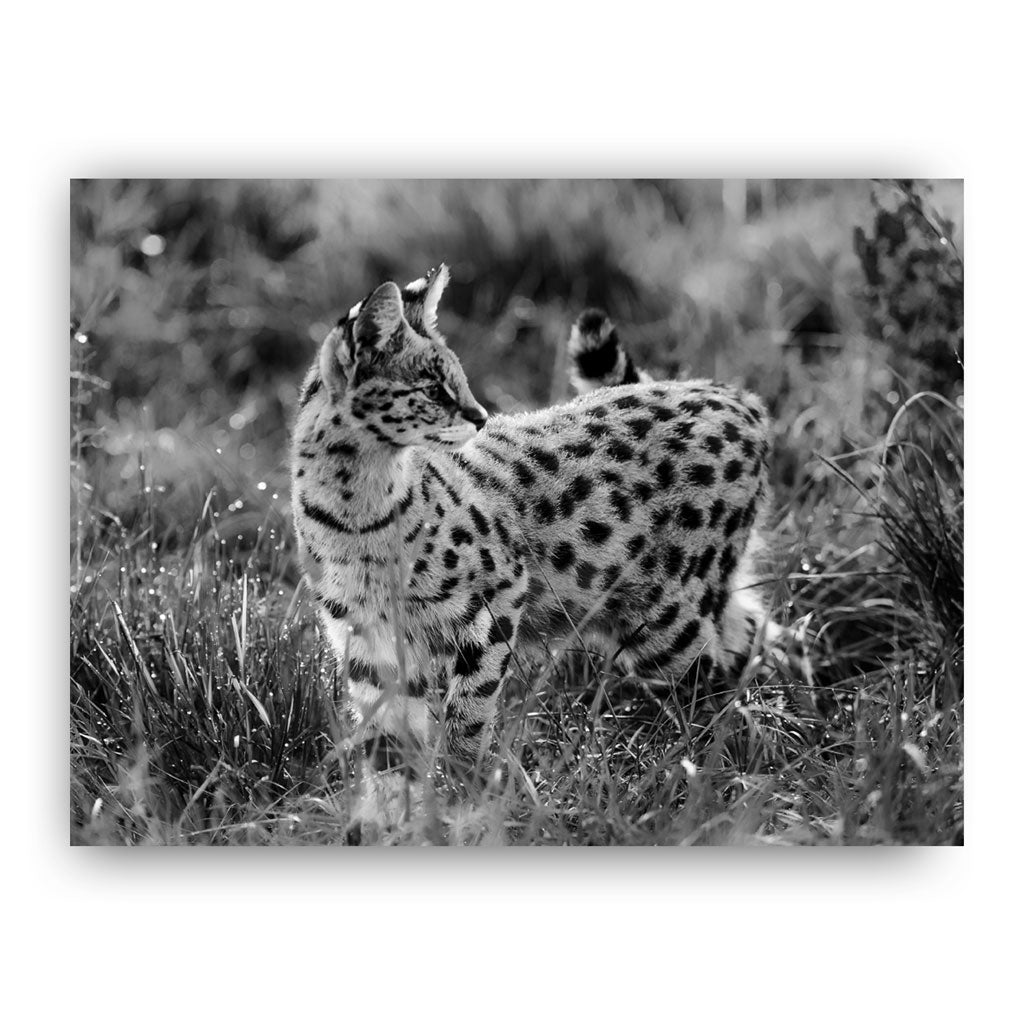This black-and-white photograph captures a young leopard standing majestically amidst dense, tall grasses. Predominantly white with striking black spots, the leopard's body faces left while its head turns back to the right, allowing a clear view of its piercing eye, which is a mix of yellow and gray hues. Its alert ears, lined with white fur, stand tall, and its black nose points downward. The leopard's tail curls gracefully over its back, marked by a distinctive black tip followed by a white and a black section. The scene is set against a completely out-of-focus, fuzzy background, emphasizing the leopard as the central focus. The surrounding grass, with sporadic white-tipped blades, suggests a savannah setting, giving the image a wild and untamed atmosphere.